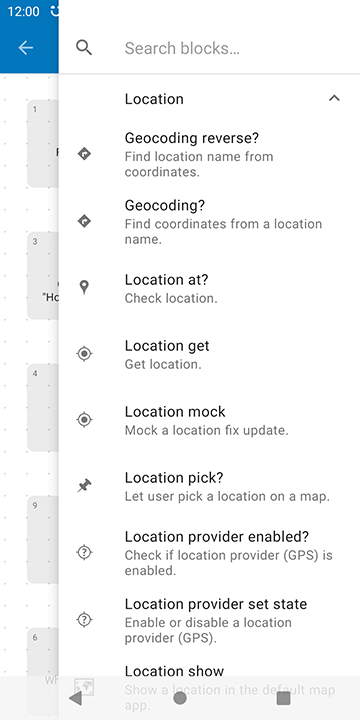This screenshot from a smartphone displays the interface of a software application with two overlapping screens against a white background. The screen in the background, positioned on the left, features a blue border at the top with the text "12 o'clock" and a left-facing arrow, likely indicating time and a navigation option. Below this, the screen has a white background adorned with small gray dots arranged in a grid pattern and five vertically aligned gray boxes.

The foreground screen on the right also has a white background at the top, featuring a search bar with a magnifying glass icon and the text "Search blocks." Beneath the search bar, a thin gray line extends horizontally across the screen, followed by the label "Location" on the left side, with an upward-facing arrow to the right, suggesting a dropdown or expandable menu.

Further down, a list of location-related options is present, each accompanied by an icon on the left. These options include:
- **Geocoding Reverse**: Find location name from coordinates
- **Geocoding**: Find coordinates from a location name
- **Location At**: Check location
- **Location Get**: Get location
- **Location Mock**: Mock a location fix update
- **Location Pick**: Let user pick a location on a map
- **Location Provider Enabled**: Check if location provider (GPS) is enabled
- **Location Provider Set State**: Enable or disable a location provider (GPS)

The descriptive icons next to each option offer visual cues for their functionality, enhancing user navigation and interface interaction.